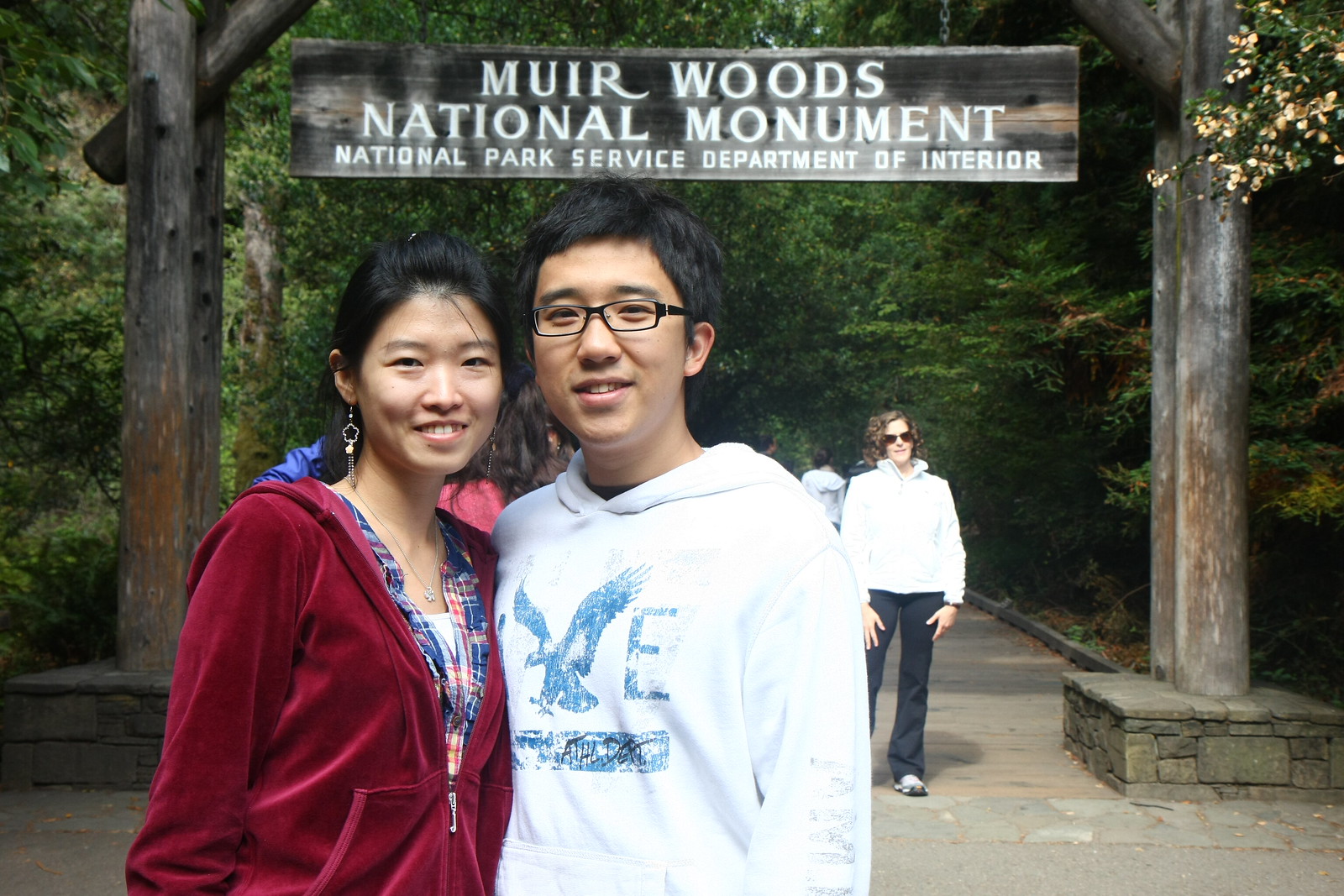In this image, two young Asian individuals, a man and a woman, are posing for a photo at the entrance of Muir Woods National Monument. They are standing under an arch made of wooden logs that supports a sign reading "Muir Woods National Monument, National Park Service Department of Interior." The young woman is dressed in a red velour jacket and the man in a white hoodie; both are wearing glasses, and the woman also has earrings. Behind them, a lush backdrop of green trees and shrubs can be seen, typical of the park's wooded area. Additionally, a woman wearing black pants, a white hoodie, and sunglasses appears to be photobombing in the background. The setting includes a well-trodden path winding through the greenery, highlighting the natural beauty of the monument. People are visible congregating in the vicinity, giving a sense of a popular, well-visited park.